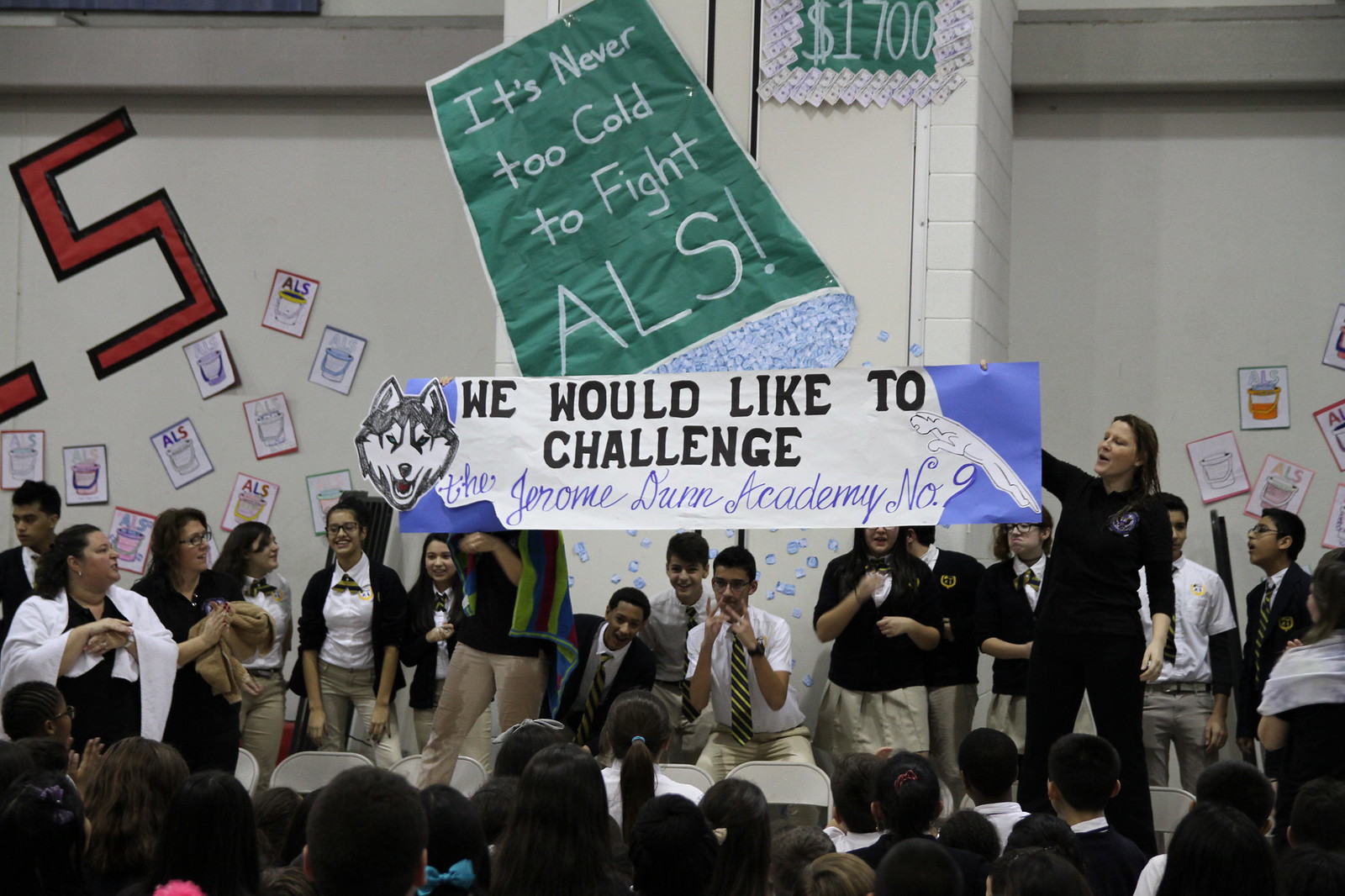The image depicts a lively school assembly, likely a pep rally or fundraiser, centered around a large-scale ALS ice bucket challenge. Students, dressed in school uniforms with black blazers, white button-up shirts, and yellow and black neckties, are gathered on a stage. Prominently displayed is a towering, six-foot-tall green paper bucket with "It's never too cold to fight ALS" inscribed in white. 

Additionally, several students hold a white banner adorned with a blue and white wolf mascot alongside a cat, challenging the Jerome Dunn Academy No. 9. The backdrop features white walls decorated with student-made posters about ALS, and a sign at the top indicating they have raised $1,700. Among the audience seated on fold-out chairs, one student is notably wrapped in a towel, reinforcing the ice bucket challenge theme. The scene is energetic and spirited, highlighting the community's dedication to raising awareness and funds for ALS.